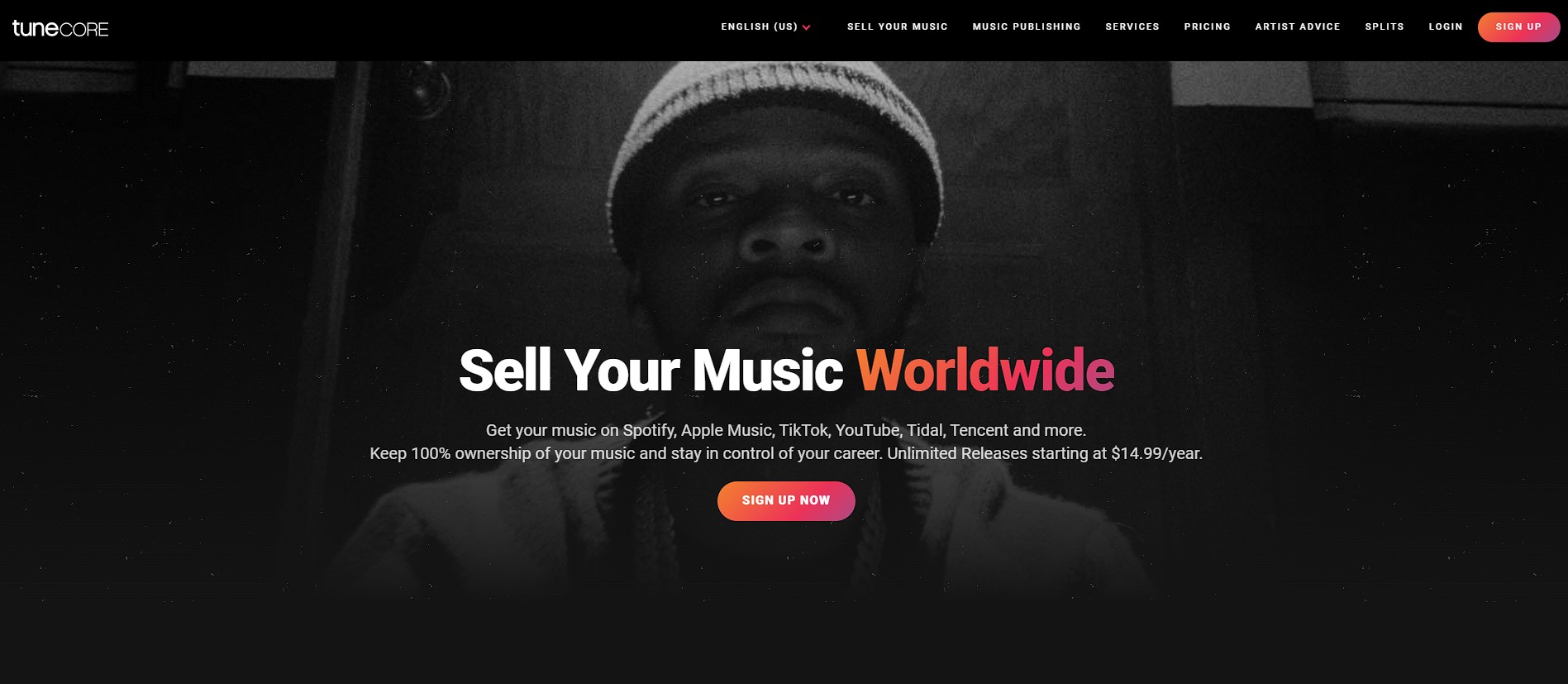### Screenshot of TuneCore Website

The screenshot captures the homepage of the TuneCore website, characterized by a modern, user-friendly design. The top section features a black navigation bar with various categories, including a language selection drop-down menu, options such as "Sell Your Music," "Music Publishing," "Services," "Pricing," "Artist Advice," "Splits," and "Login." At the far right of the bar, there is an eye-catching gradient button transitioning from orange to pink labeled "Sign Up."

Dominating the screen is a large black-and-white photograph of a young Black man, approximately 30 years old. He has a thin mustache and beard, and he's wearing a beanie hat. His attire includes a cloth-looking jacket, contributing to a casual, yet professional vibe. 

Superimposed on the image, in stark white text, is the phrase "Sell Your Music," followed by "worldwide" in a gradient transitioning from orange to pink. Below this headline, it encourages artists to get their music on major platforms such as Spotify, Apple Music, TikTok, YouTube, Tidal, Tencent, and more, all while retaining 100% ownership and control of their careers. The text further highlights the start price, "Unlimited releases starting at $14.99 a year."

Towards the bottom, a small, prominent button, in the same orange-to-pink gradient, urges visitors to "Sign Up Now." The background of the image shows a door and wall, with a door handle visible above and to the left of the man, adding an element of depth and context to the scene.